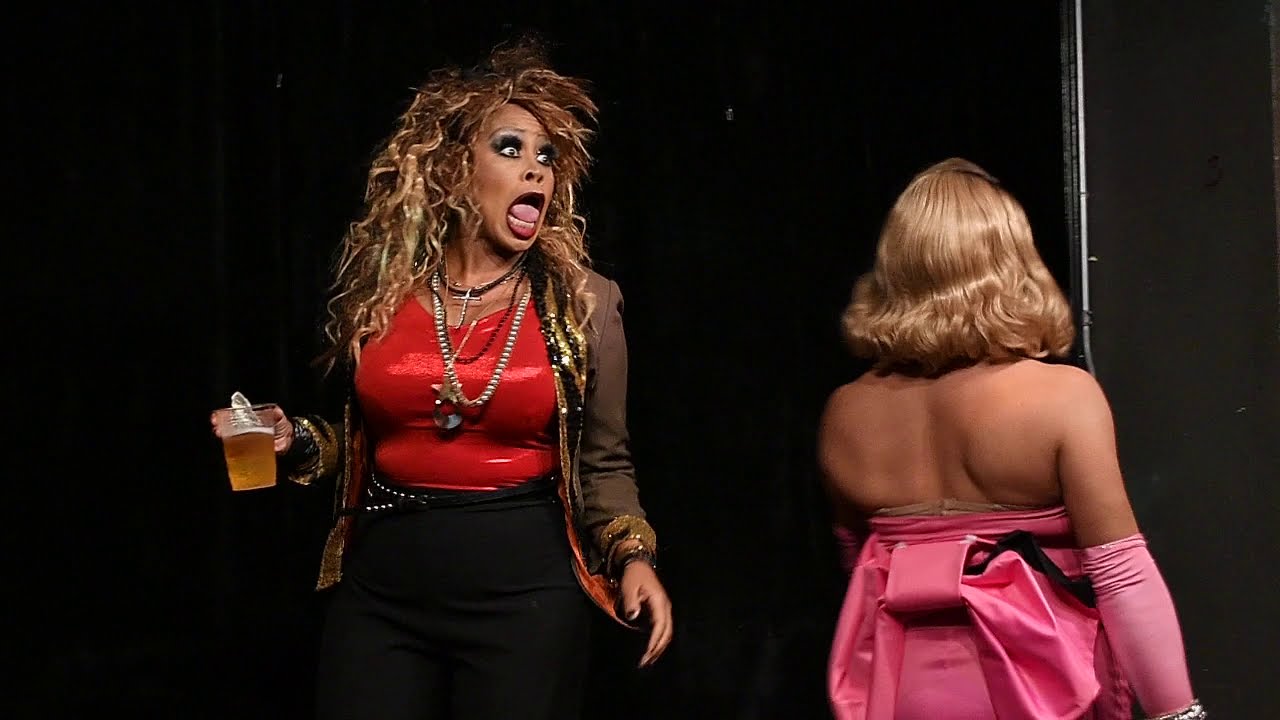This photograph features two women set against a predominantly black background. The woman on the left, with long, squiggly, blonde-highlighted hair, appears vibrant and animated, as she loudly screams with her mouth wide open, revealing her tongue and bottom teeth. Her elaborate makeup complements her striking outfit—a red tank top beneath a brown long-sleeved coat, paired with black pants. She accessorizes with several necklaces, including one with a cross, and flaunts long nails. In her right hand, she holds a clear glass filled with a foamy yellow beverage, likely beer. Her left hand rests lower, down by her side. Beside her, the second woman, positioned to the right, shows only her back to the camera. She sports short blonde hair, possibly a wig, which curls slightly at the ends. She wears an elegant, backless pink dress paired with long pink elbow gloves. A slight patch of gray can be seen to the right, breaking the otherwise all-black background.